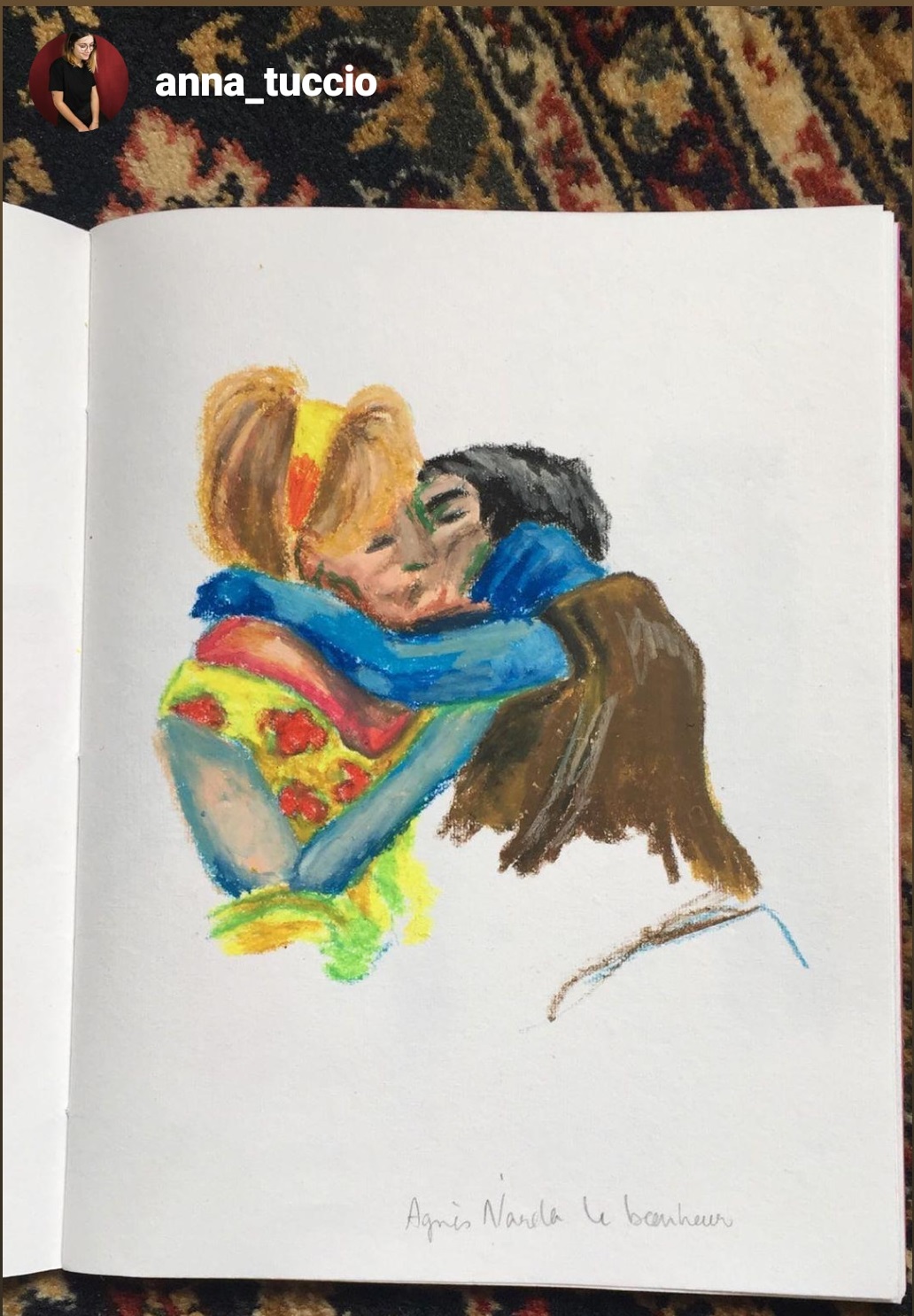Here is a detailed and descriptive caption for the given Instagram post:

---

In this colorful Instagram post, user "anna_tuccio" shares a stunning pencil sketch from her vibrant artist's drawing book. The sketch, immaculately detailed, features two people in a tender embrace. The woman, with shoulder-length blonde hair adorned with a yellow and red headband, is captured in a moment of affection. She wears a dress adorned with red roses, accompanied by a red scarf or collar, creating a harmonious blend of colors. Her eyelids gently closed, she is seen kissing a person with short black hair. This individual, clad in a blue scarf and a brown shirt, also has their eyes shut, capturing the sincerity of the moment. The drawing's lower right corner shows traces of the artist's signature on a white background, though the full signature remains unreadable. Anna's meticulous use of color and detail brings this intimate scene to life, painting a picture of pure emotion and artistry.

---